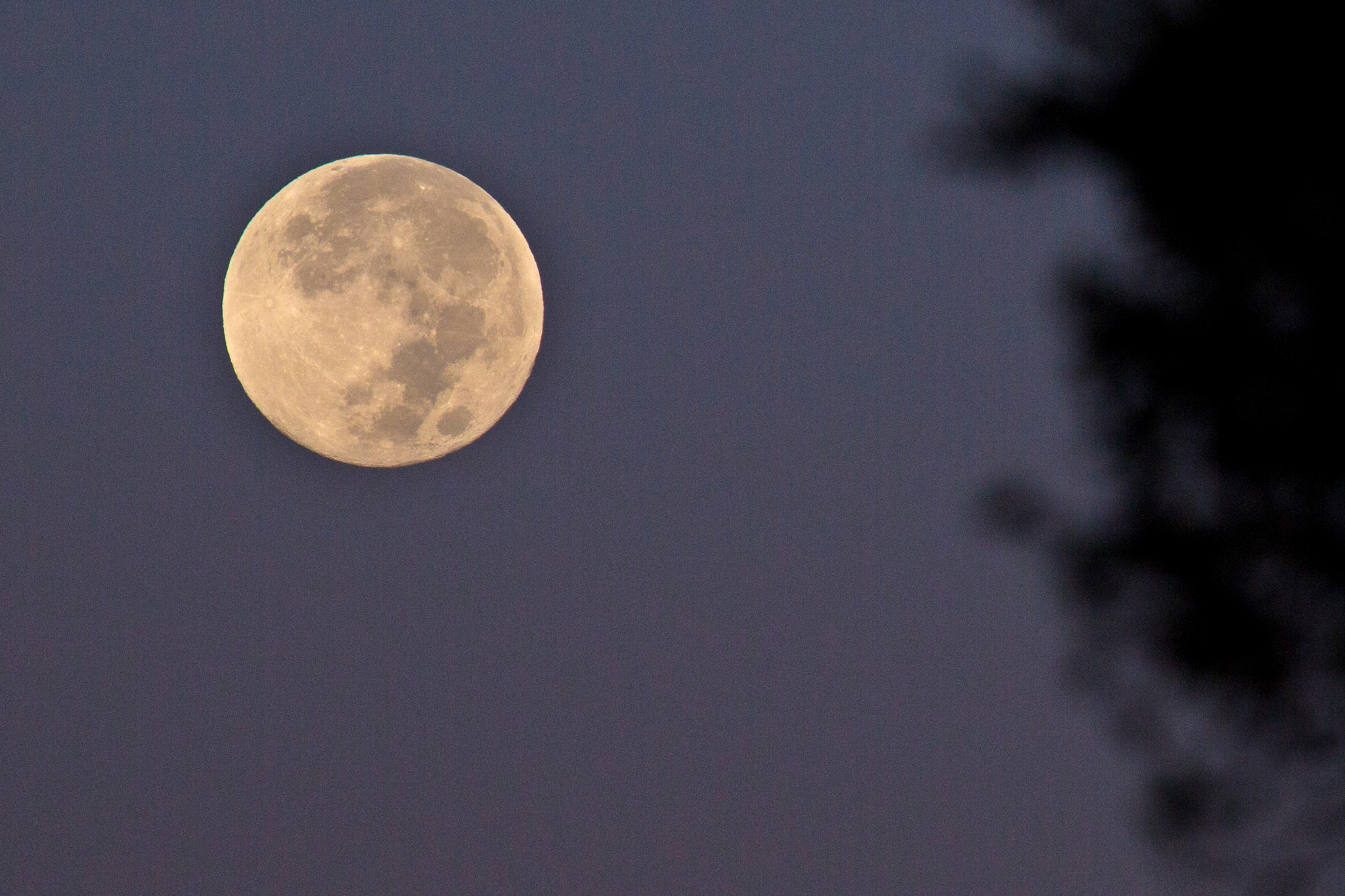A full moon glows with a light yellow and orangish hue, prominently positioned in the top left of the night sky. The moon's surface reveals detailed shading from large craters, with the right side particularly craggy in appearance. The rest of the sky transitions through shades of dark grayish-blue and light blue-gray, suggesting it’s shortly after dusk. On the right, a silhouette of blurred trees or bushes stretches from the top right to the bottom right of the image, framing the celestial scene. The sky is clear, devoid of any clouds, allowing the moon to shine brightly and uninterrupted.